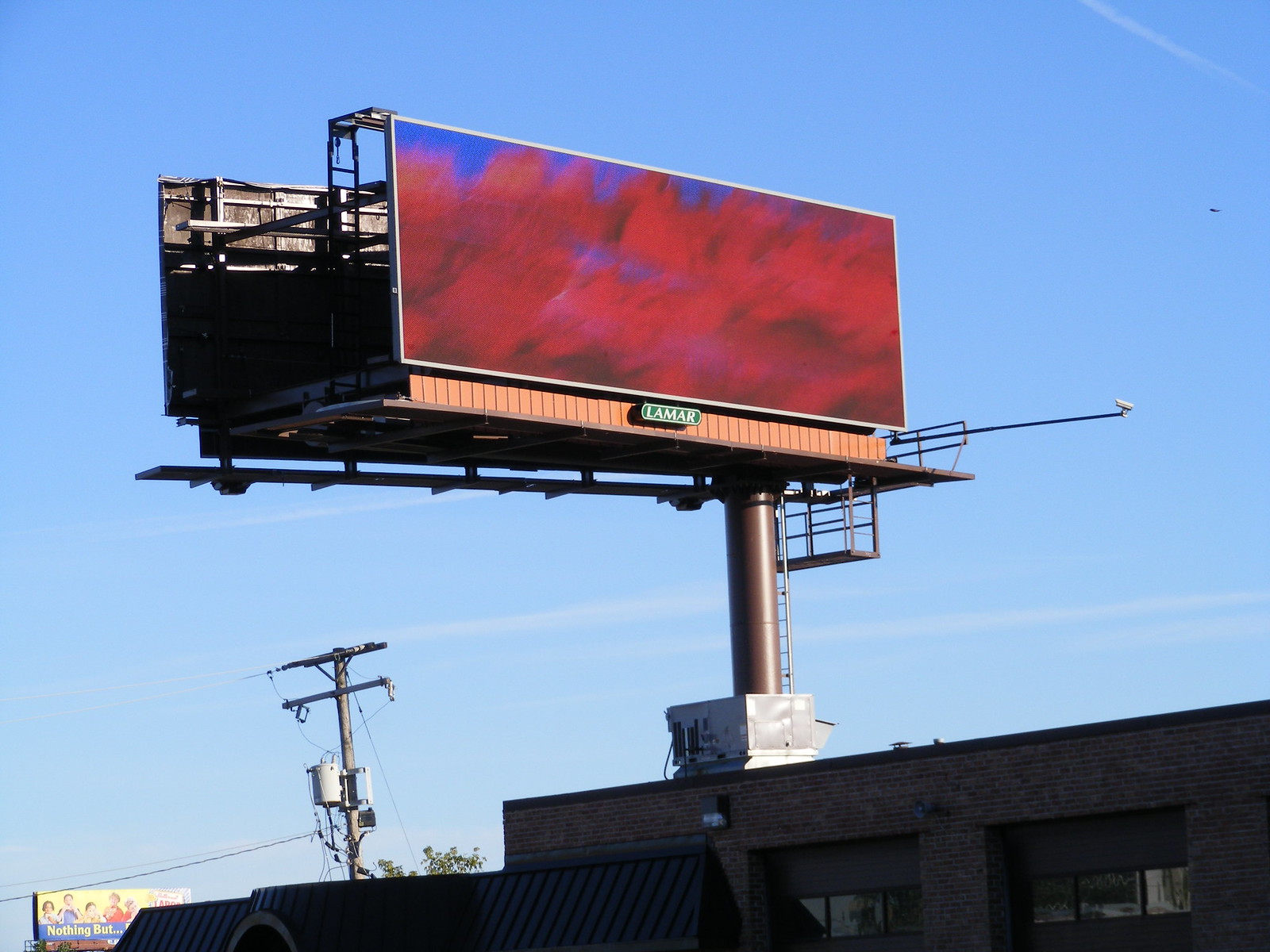The image showcases a prominent billboard perched atop a gray building against a vibrant blue sky. To the left of the billboard, several telephone poles are visible, adding an urban element to the scene. The billboard itself is mostly blue with some red accents, and features a green segment with the brand name "Lamar" displayed on it. Beneath this, there are slats in a mix of orangey and pinky hues. The structural supports of the billboard are made of silver metal, gleaming under the bright daylight. The color palette of the image includes shades of gray, blue, red, light blue, white, silver, and hints of orange and pink, creating a visually engaging contrast. The purpose of the billboard remains ambiguous as it does not convey any specific message.